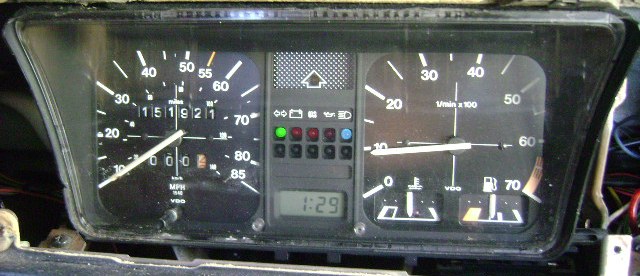This close-up photograph captures the dashboard of a motorized vehicle, prominently featuring two gauges. On the left, a speedometer is displayed, which measures the vehicle’s speed up to 85 miles per hour. In the center of the speedometer, the odometer reads 151,921 miles, indicating the total distance the vehicle has traveled. The speedometer needle, used to indicate the current speed, is colored white for easy visibility.

On the right side of the dashboard, there is another gauge that seems to measure either fuel levels or engine RPMs, marked from 10 to 70 in increments of 10. Positioned in the middle of the dashboard is a digital clock with a grayish-green background, showing the time as 1:29, though it does not specify whether it is AM or PM.

Above the clock, a row of indicator lights is visible, designed to alert the driver to various vehicle issues. These indicators include symbols for headlights, battery, and other essential vehicle functions. The overall composition of the photograph focuses on these critical dashboard elements, providing detailed insight into the vehicle's instrumentation.